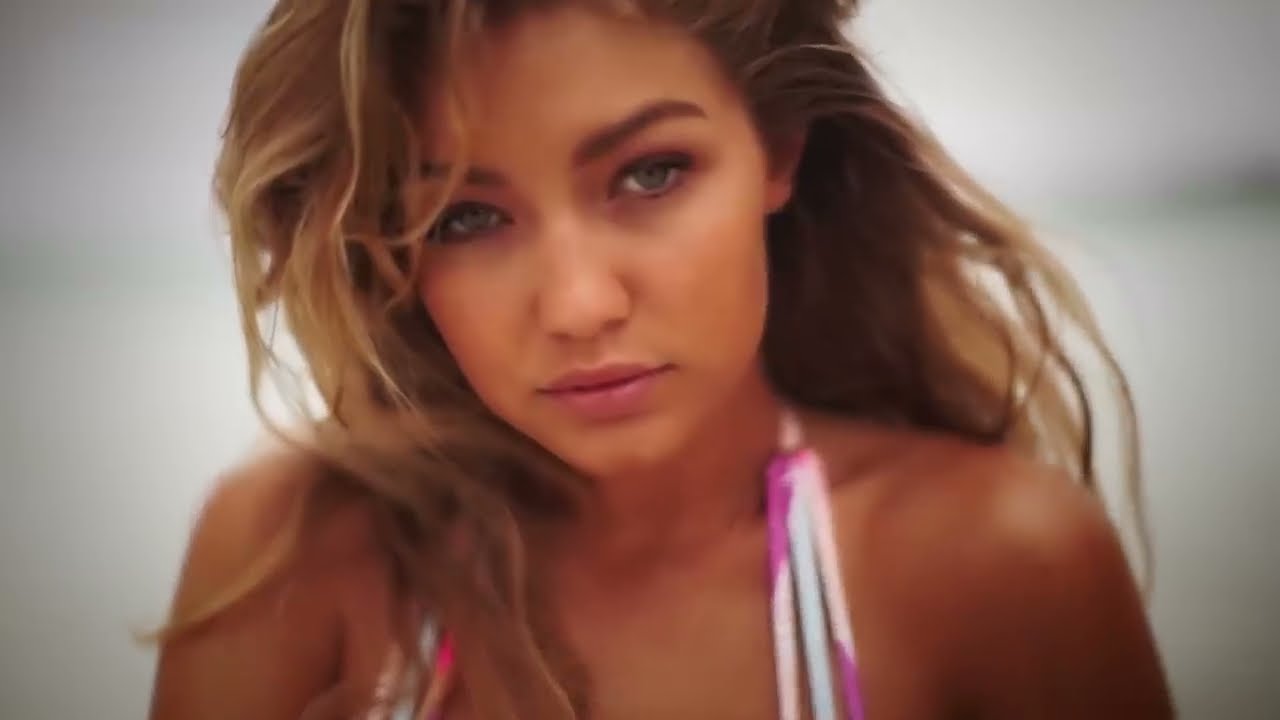In this slightly blurry and possibly outdoor photograph, yet suggesting a studio setting, we see the famous model Gigi Hadid. Portrayed in a summery vibe, Gigi's hair is styled down, slightly tousled by the wind, enhancing her casual, carefree look. She has a tanned complexion, whether naturally sun-kissed or influenced by the lighting, which gives her an orangish glow. Her makeup is light and natural, with a touch of pink lipstick giving her a fresh, summery charm. Gigi's piercing green eyes, framed by brown eyebrows, are directed straight at the camera, and her head is slightly tilted, adding a subtle depth to her gaze. She is wearing a strappy halter bikini top in shades of white and pink that hints at a playful, beach-ready fashion, despite only the straps being visible in the image. The backdrop is notably blurred, highlighting Gigi as the central focus and creating a contrast between her vibrant presence and the muted, off-white, gray, and tan tones that form the indistinct background. The overall composition and styling suggest the photo could be a professional modeling shot aimed for a magazine spread.